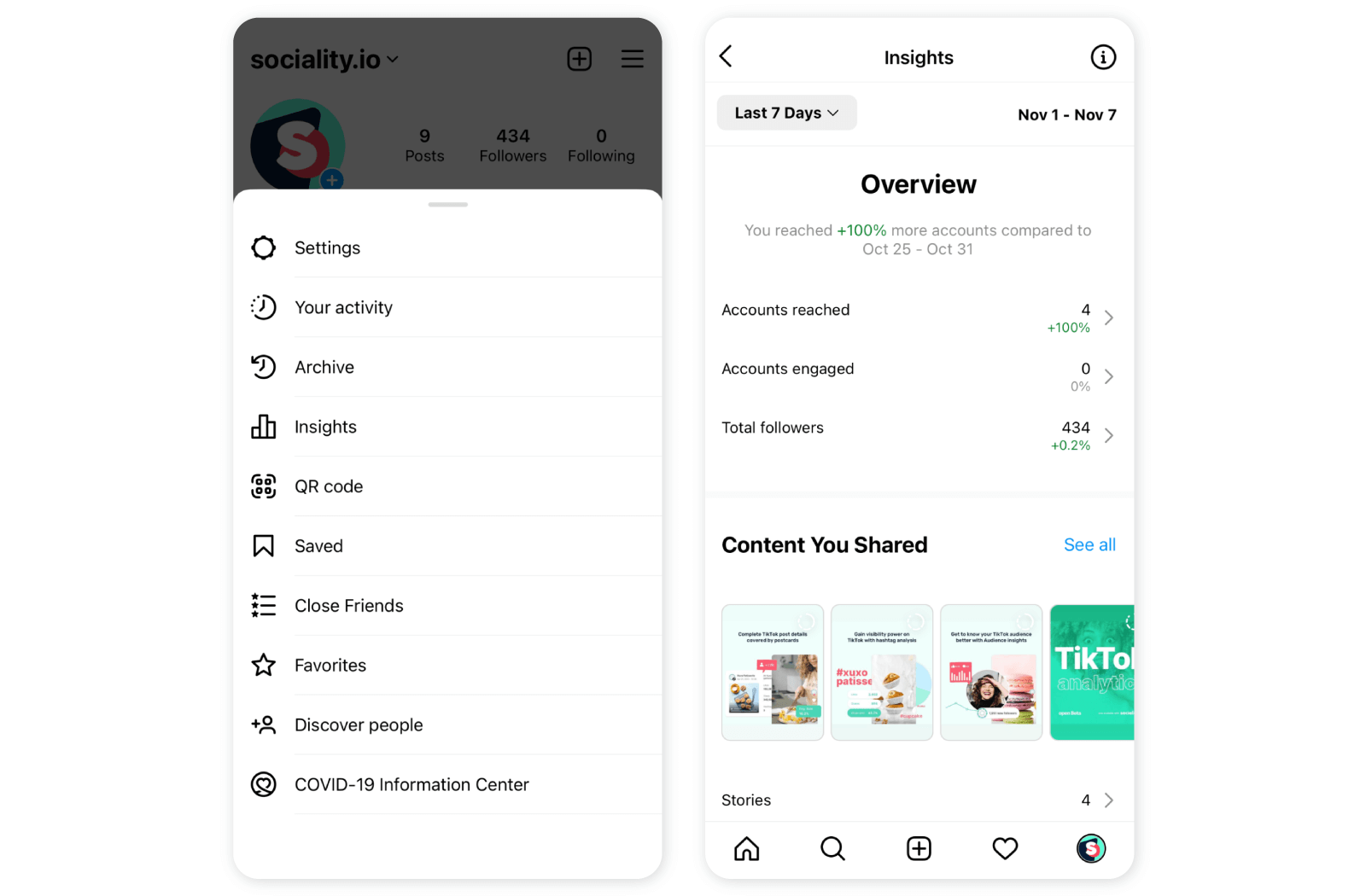Here are two side-by-side mobile screenshots of an Instagram profile analysis, featuring detailed insights into user activity.

On the left screenshot:
- It displays the top section of the Instagram profile, with the username positioned at the top left: "sociality.io".
- Below the username, there is a profile picture featuring a white 'S' on a black and green background.
- Displayed underneath the profile header are various navigation and settings options: "Settings, Your Activity, Archive, Insights, QR Code, Saved, Close Friends, Favorites, Discover People, COVID-19 Information Center".

On the right screenshot:
- Titled "Insights", it presents an overview of the profile’s performance over the "last seven days" (as indicated by the dropdown menu).
- The summary shows significant engagement metrics, highlighting that the profile "reached 100% more accounts compared to October 25 through October 31".
- The specific figures include:
  - "Accounts Reached: 4", indicating a 100% increase.
  - "Accounts Engaged: 0".
  - "Total Followers: 434".